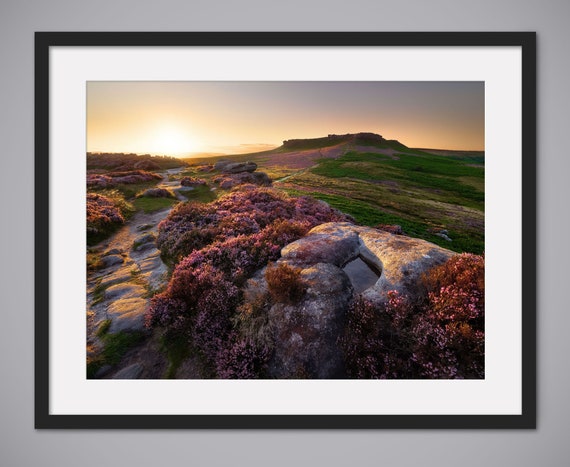The photograph captures a stunning hand-drawn landscape painting of a serene countryside at sunset, framed in a plain black frame with a white matte border. Hanging on a light gray wall, the artwork depicts an expansive, blissful scene filled with vibrant greens and lush vegetation, detailed with various colorful leaves and flowers in shades of oranges, pinks, and reds. In the foreground, a prominent grayish rock is adorned with clusters of pink and red flowers, while smaller white rocks are scattered on the left side, suggesting the remnants of a river stream. The sun sets brightly in the background, casting a warm glow over the plants and grasslands. To the right, a hill slopes gently into a valley towards the setting sun, adding depth and tranquility to the composition. The sky fades from a clear blue at the top to a warm, orange-yellow hue as it meets the horizon, perfectly encapsulating the peacefulness of this countryside scene.